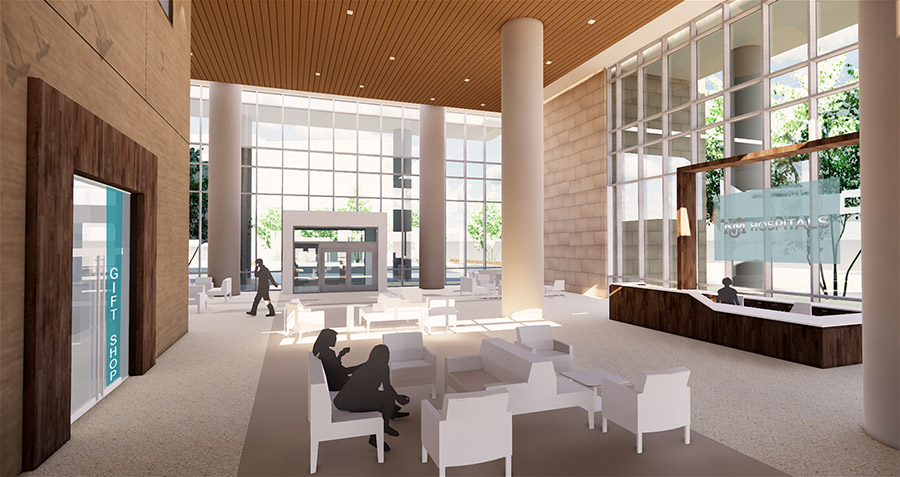The image depicts a spacious and luxurious lobby, likely part of a high-end hospital or possibly a hotel, characterized by its grand architectural features and meticulous design. At the far end of the room, the entrance is marked by electric-opening doors flanked by two tall white pillars, creating an inviting entryway. On the right side, a large, wood-paneled reception desk with white trim is attended by a receptionist. Above the desk hangs a light blue sign with grey lettering that reads "Hospitals," indicating its purpose. 

The lobby features a high, dark brown ceiling with recessed lighting and a floor that alternates between beige and gray tiles. The space is further adorned with four high pillars, supporting the expansive structure. Toward the center, white sofas and armchairs provide seating, where two silhouetted figures are visible. Nearby, one person is seen talking on the phone while walking away from the scene, adding a touch of human activity to the lobby.

On the left side of the image, a gift shop is visible, marked by a doorway with brown paneling, a white, see-through door, and a blue strip with white lettering that reads "Gift Shop." The overall color palette of the lobby includes various shades of brown and white, creating a warm and welcoming atmosphere.